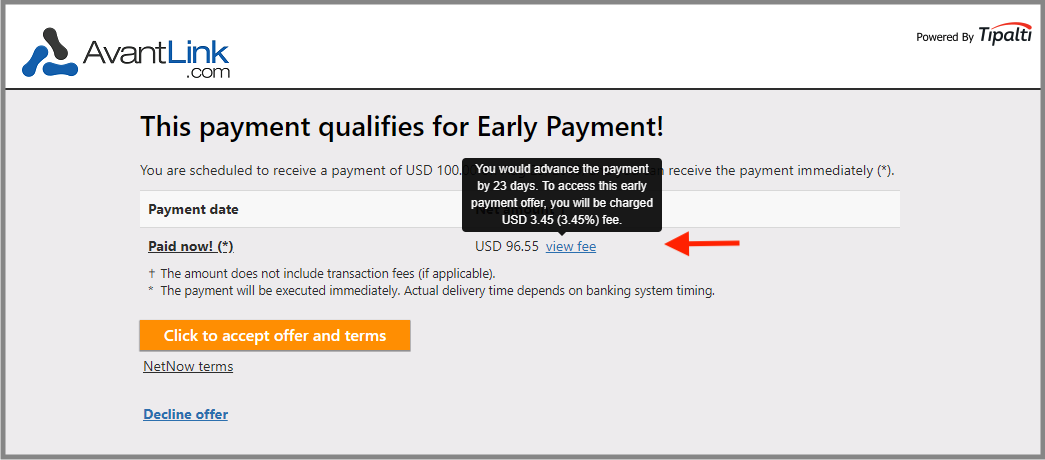The image features a detailed payment notification interface. At the top of the image, there's a white border. On the left side, there's an indistinct logo with two dark blue symbols resembling bones, accompanied by a similar black symbol. To the right of the logo, the text reads "eventlink.com," and further right, it says "powered by Tipalti."

A thin black line runs horizontally from left to right, dividing the upper section from the content below. Beneath this line, on a light gray background, a bold black heading states, "This payment qualified for early payment." After a space, a non-bold black text follows, reading, "You're scheduled to receive the payment of USD 100."

Part of the text is obscured by a black rectangle. To the right of this box, it says, "Receive the payment immediately*," with an asterisk in parentheses. The black rectangle contains white text explaining, "You would advance the payment by 23 days. To access this early payment offer, you will be charged a 3.45% fee (USD 3.45)."

Below this explanation, a red arrow points downward towards the text "USD 96.55," indicating the net amount after the fee is deducted. To the left of the red arrow, the phrase "View fee" is displayed.